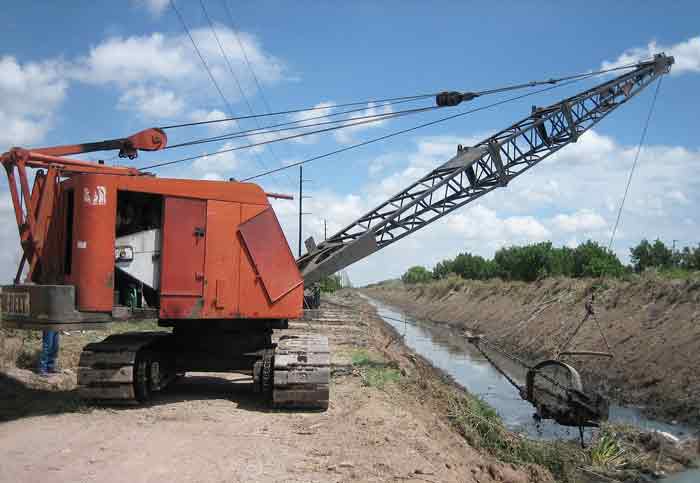The photograph captures a scene of a large, square-shaped piece of machinery, colored in shades of orange and red, working outdoors under a blue sky with puffy white clouds. The equipment, resembling both a crane and farm machinery, is positioned on tank-like tracks and slants slightly forward. It is operating on the bank of a long, narrow waterway, which is flanked by brown, muddy dirt mounds. On the right side of the image, there is a stretch of green trees. The machinery has an extended black crane arm reaching into the water, appearing to lift a metal and muddy object. A panel on the machine is open, revealing some internal mechanical parts. Additionally, a pair of legs in blue jeans, belonging to a man whose upper body is obscured by the equipment, can be seen behind the machine. The setting conveys a robust and industrious scene, likely involving the extraction or movement of materials from the waterway.